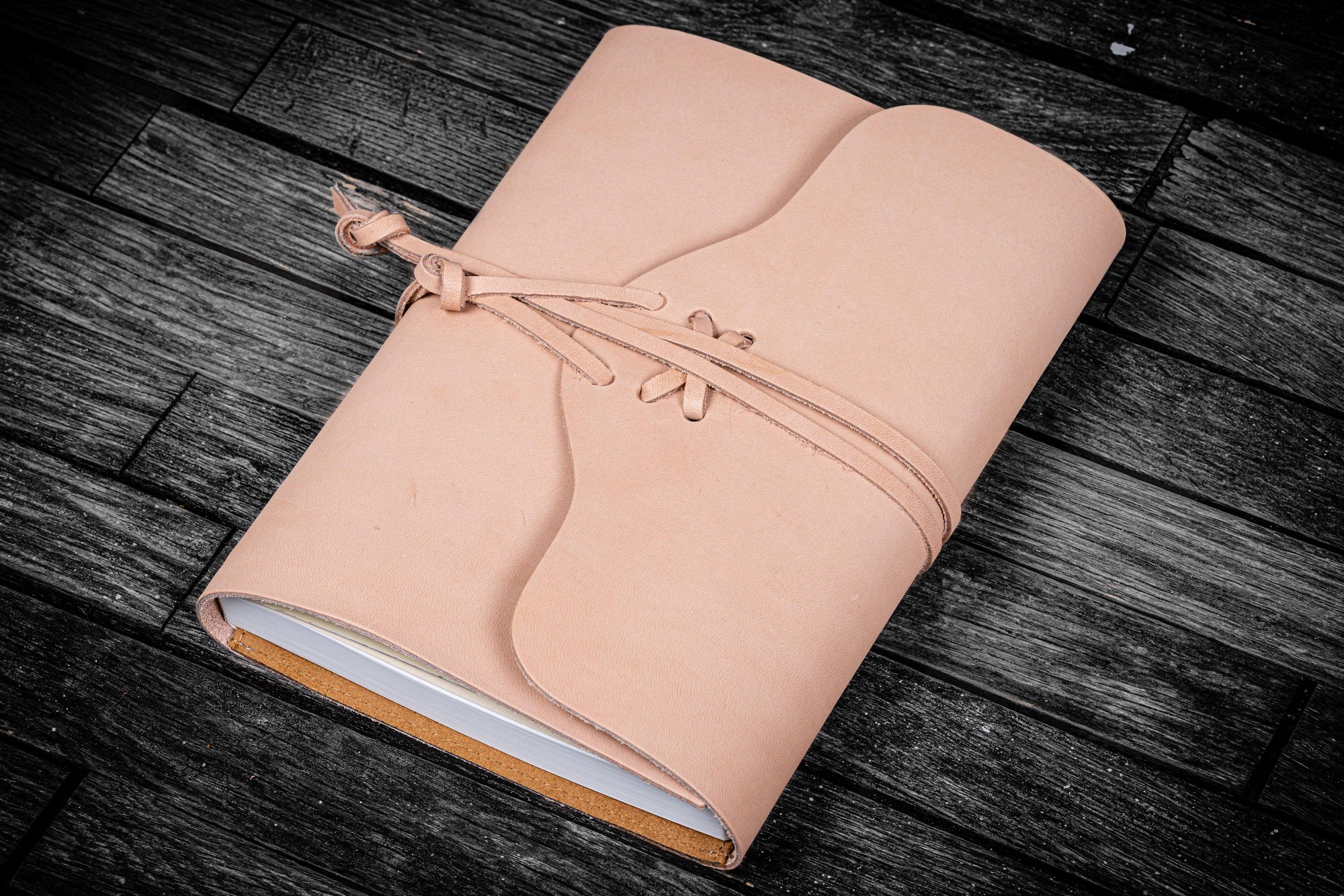This is a close-up, angled view of a leather-wrapped journal resting on a dark wooden table with small grayish-black planks. The journal is made of pink, or a light pinkish-coral colored, leather and features an envelope-style closure. It is secured with two leather ties that are intricately knotted at the front, forming a small leather 'X' on the surface. The journal has a scalloped-edge design that wraps around like a package, revealing a glimpse of the tan leather interior beneath the edges of the white paper inside. This detailed and stylish accessory could serve various functions, possibly holding note paper or even an e-reader, set against the richly textured wooden backdrop.